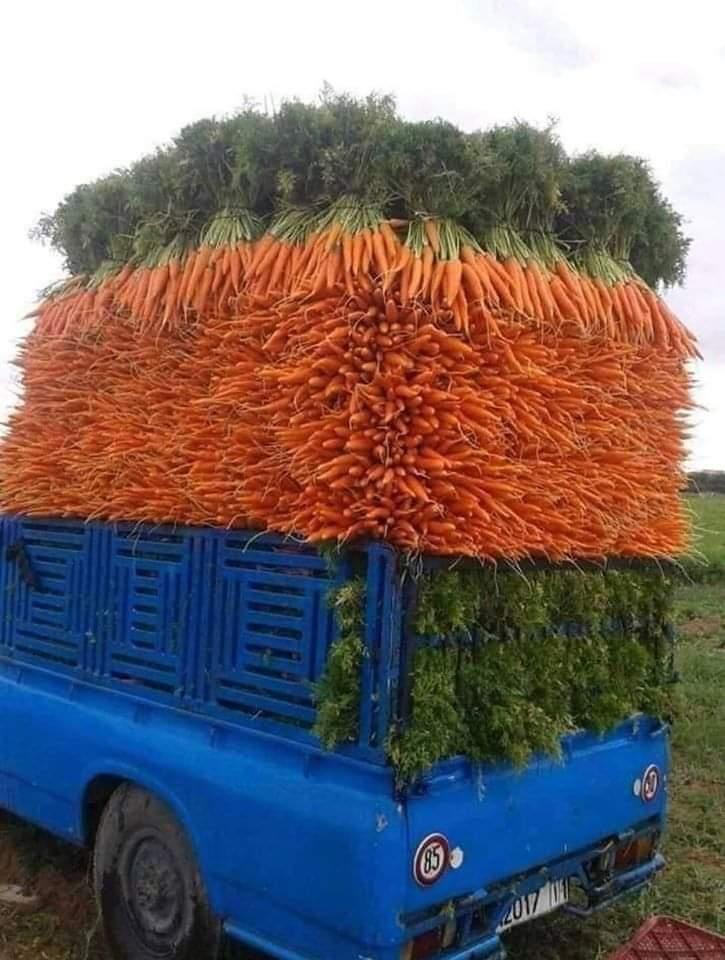The image shows a bright blue truck loaded with a gigantic stack of freshly picked, vibrant orange carrots. The carrots, arranged in a uniform and perfectly rectangular bundle, are piled high, extending twice the height of the truck itself. The bundle creates a pyramid-like structure, with the bushy green tops of the carrots spilling out above. Some of the wire can be seen securing the greenery at the top, adding an interesting texture to the scene. Below and around the carrots, parts of the truck bed and paneling are visible, with additional carrot tops protruding through. The truck's back features two prominent circles with the number 85, and a grassy field stretches out on the right side of the image. Despite the neatly stacked appearance, it seems as if any forward motion could easily cause the massive haul to topple over.